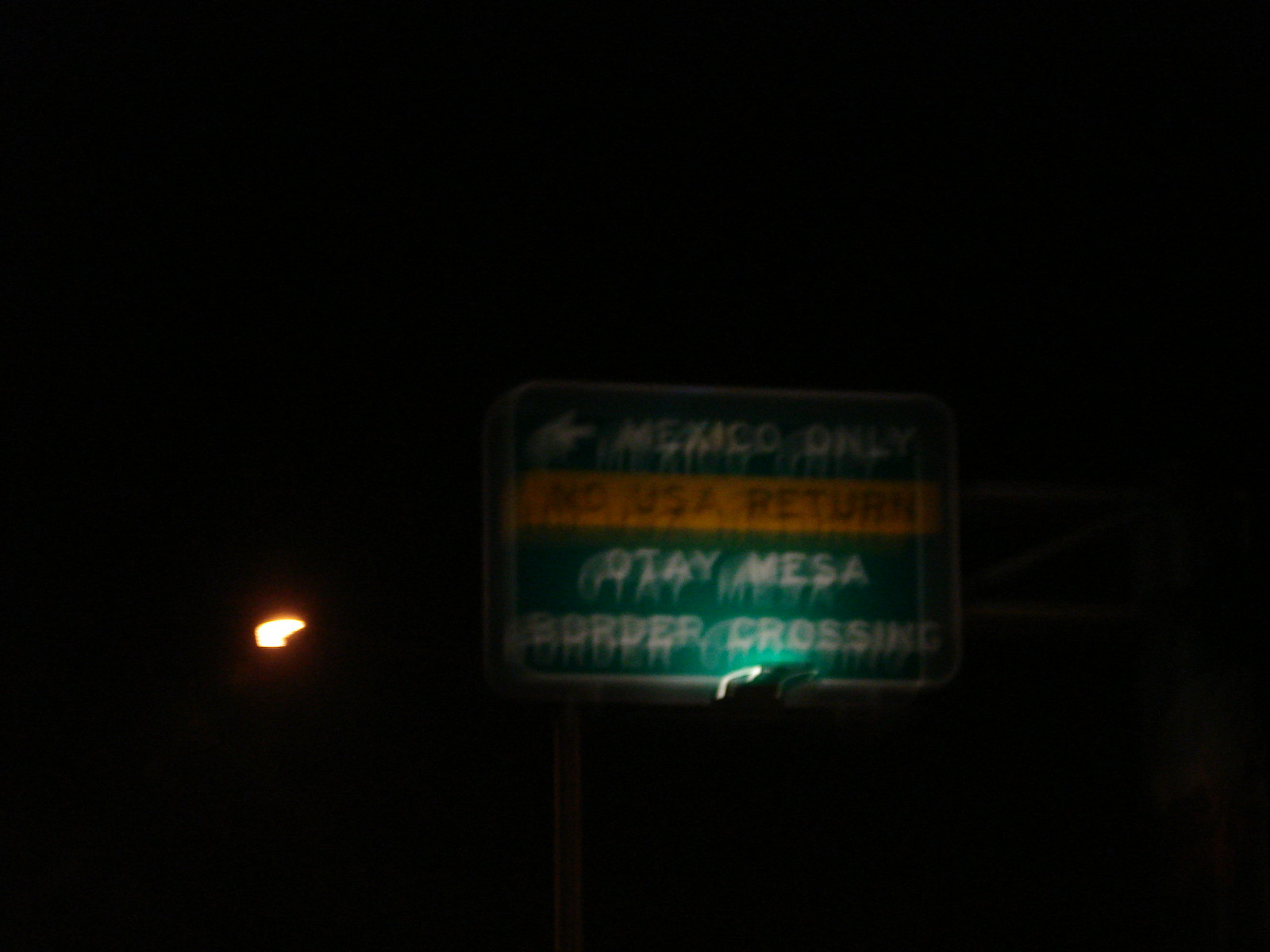This night-time photograph captures an illuminated green road sign, typically found on freeways or at airports. The sign, outlined in white, prominently displays the words "MEXICO ONLY" in capital white letters accompanied by a left-pointing arrow. Below this, a distinct orange horizontal stripe bears the text "NO USA RETURN" in black, also in uppercase. The third line reads "OTAY MESA," and the final line states "BORDER CROSSING," both in white, capital letters. The background of the image is pitch dark, intensifying the glow of the lamppost positioned to the left of the sign, casting light in the surrounding darkness.